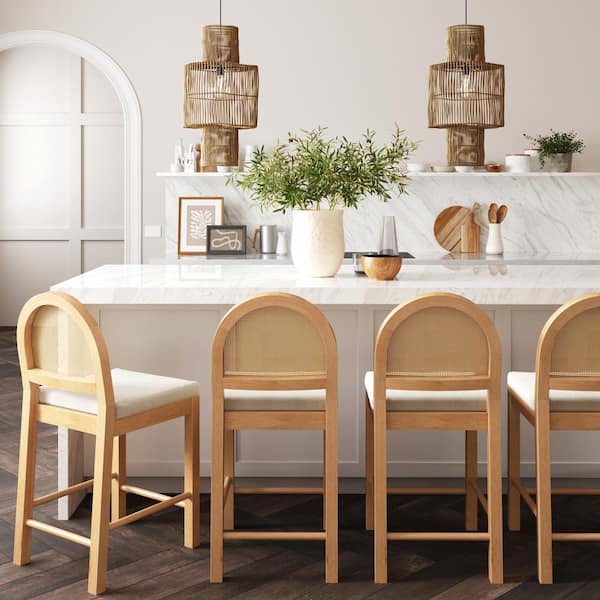This image showcases a meticulously staged dining area that could also function as part of a kitchen, perfect for advertising furniture or kitchen setups. Dominating the space is a central island featuring an exquisite white marble countertop and backsplash. Atop the marble surface, a potted plant in a white circular planter, several wooden bowls, plates, a few framed pictures, and small utensils are meticulously arranged. The backdrop is a pristine white wall, contrasting elegantly with the dark hardwood flooring.

Prominently featured are four high bar stools with a blondish light wood finish and white square cushions, each with a small curved wooden back. Only one stool is slightly angled, adding a touch of realism to the otherwise meticulously arranged scene. Above, two wicker or bamboo lantern-style lamps provide a rustic charm and soft illumination.

To the left, a curved entryway arch subtly transitions into the next room, enhancing the open and airy feel of the space. This expertly staged photo elegantly captures a harmonious blend of modern and rustic elements, making it ideal for showcasing home furniture and kitchen designs.